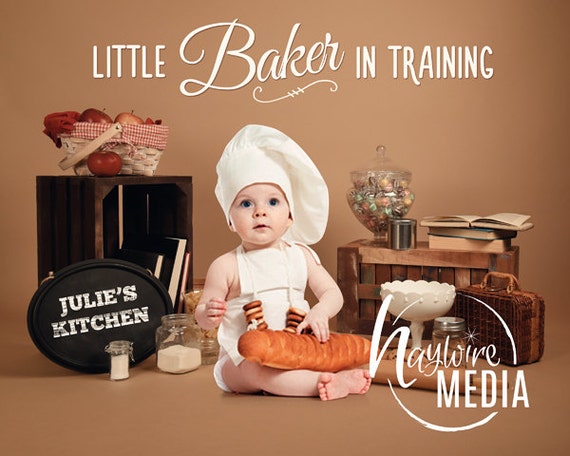The advertisement poster features a cute baby dressed as a baker, wearing only a chef's hat and a white apron, sitting cross-legged with a loaf of bread on his lap and a stack of cookies nearby. The background is predominantly brown, providing a warm, rustic feel. Above the baby, in white text, it reads "Little Baker in Training." At the bottom right corner, there is the label "Haywire Media" encircled partially, also in white text.

To the right of the baby, a sign in white text against a black circular background reads "Julie's Kitchen." Behind the baby, there is a wooden crate standing on one end, containing a basket of apples on top and some lined-up books at the bottom. Another wooden crate, placed upside down and used as a table, holds a tall vase filled with candy. Scattered around are various kitchen items, including three glass jars filled with different powdery substances and a rolling pin on the ground next to the baby. Three stacked books and additional kitchen paraphernalia complete the cozy, culinary setting.